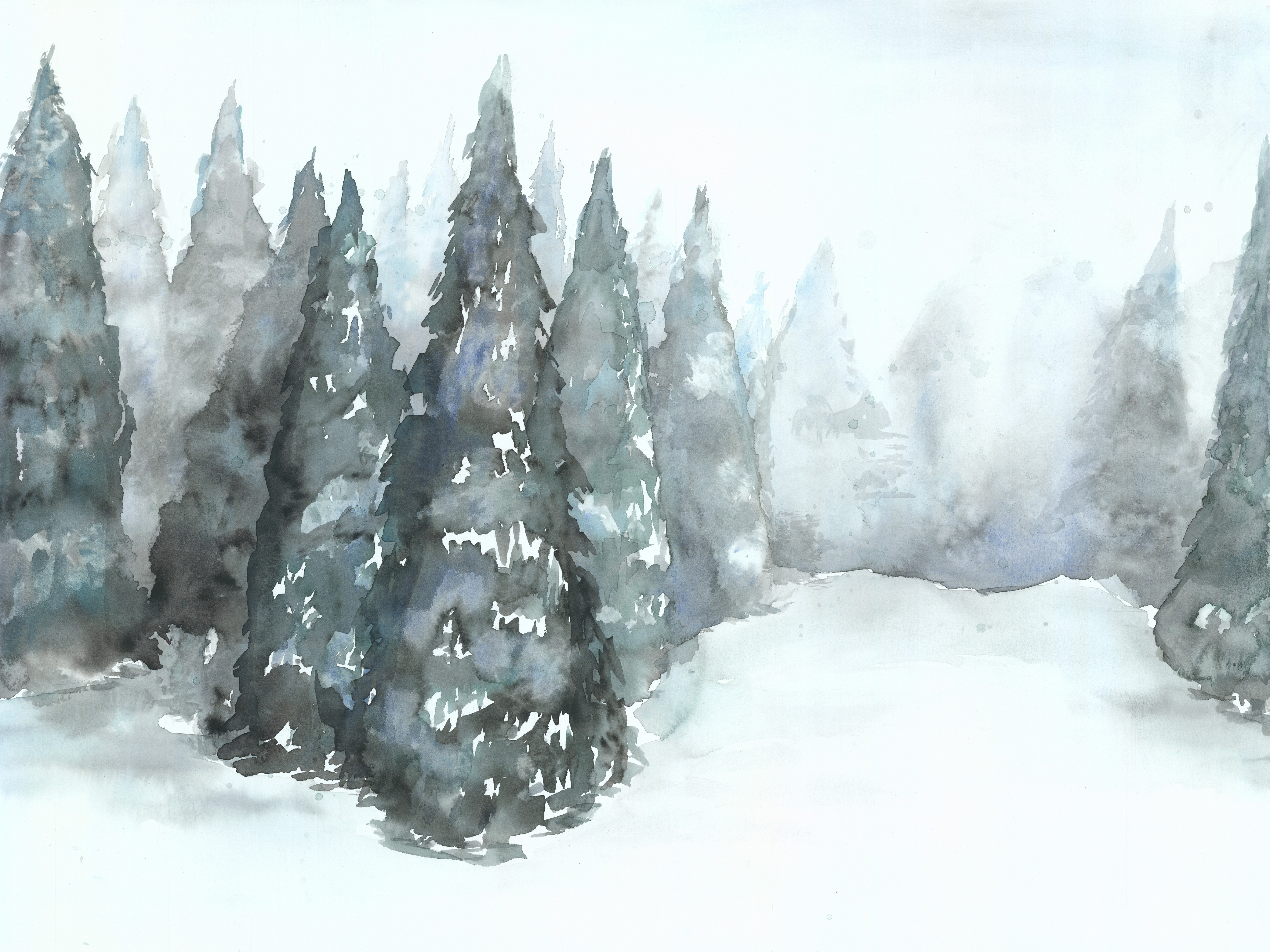This image depicts a watercolor painting, potentially created with digital tools, capturing a serene winter scene of a pine forest blanketed in snow. The painting primarily features a series of conical, dark green trees that are scattered across the snow-covered ground. The trees in the foreground are more distinct and detailed, with visible patches of snow on their branches. As the rows of trees retreat into the background, they become increasingly hazy, shrouded by an enveloping fog or perhaps a fine winter mist, which lends an ethereal quality to the scene. The sky overhead is overcast, contributing to the muted, grayscale tones that dominate the painting, enhancing the overall sense of a quiet, foggy winter day.